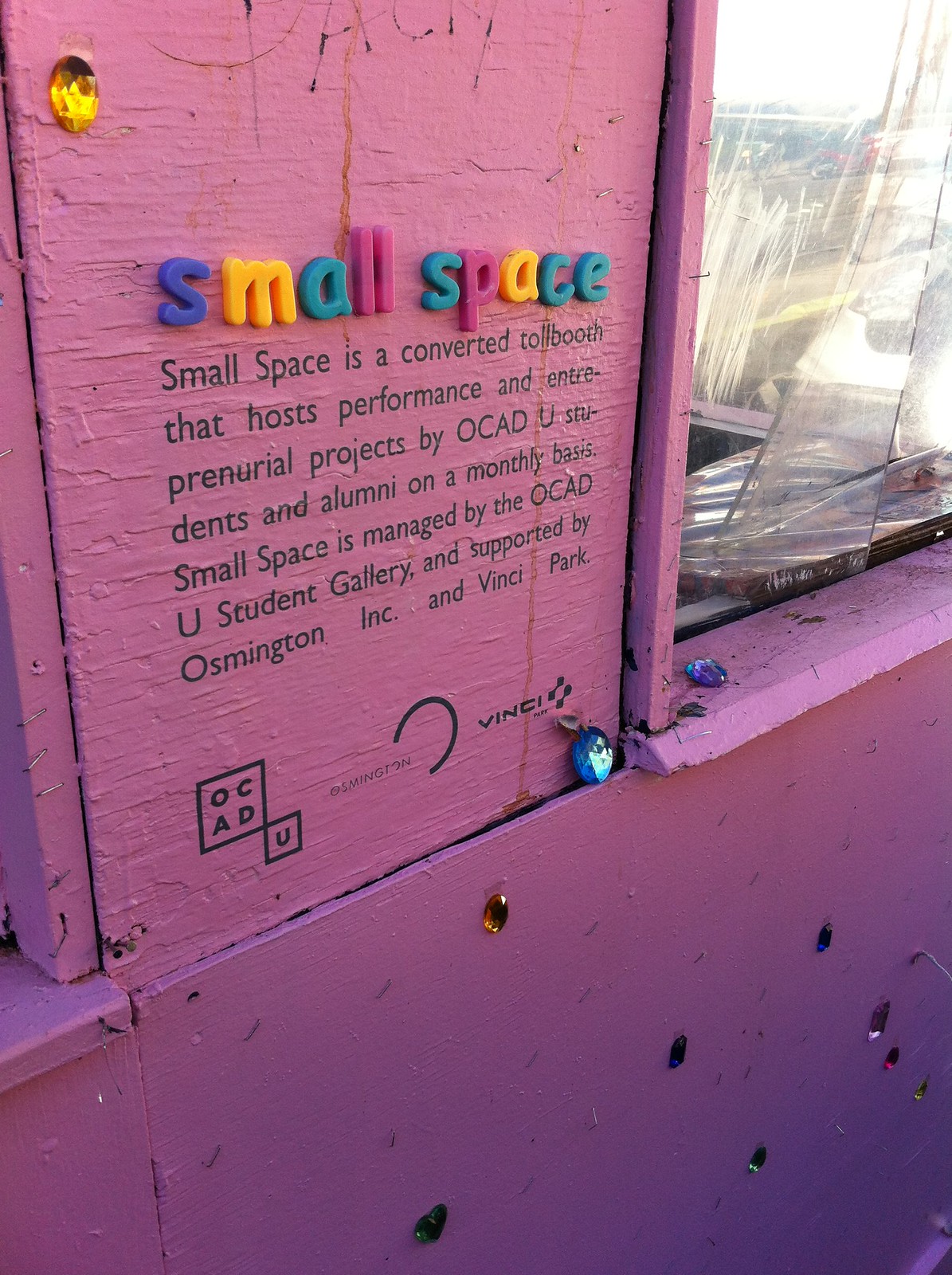This image depicts the side of a painted purple wooden structure, possibly a converted toll booth, adorned with various objects and text. In the upper third of the image, there's a window on the right, with another window partially visible on the left side of the frame. The primary feature on the wall is the phrase "Small Spaces" spelled out in colorful magnetic letters, with each letter in a different color: S (purple), M (yellow), A (blue), LL (red), S (blue), P (pink), A (yellow), and CE (blue-green). Below this in black ink, it reads: "Small Spaces is a convention toll booth that hosts performing and entrepreneurial projects by OCAD U students and alumni on a monthly basis. Small Spaces is managed by the OCAD U Student Gallery and supported by Osmington Incorporated and Vinnie Park." Beneath this text are icons representing Vinnie Park and OCAD U. The wall features small decorative jewels in green and orange, glued intermittently around the lettering. The scene appears to be outdoors, in daylight, showcasing a blend of creative elements and informational content.